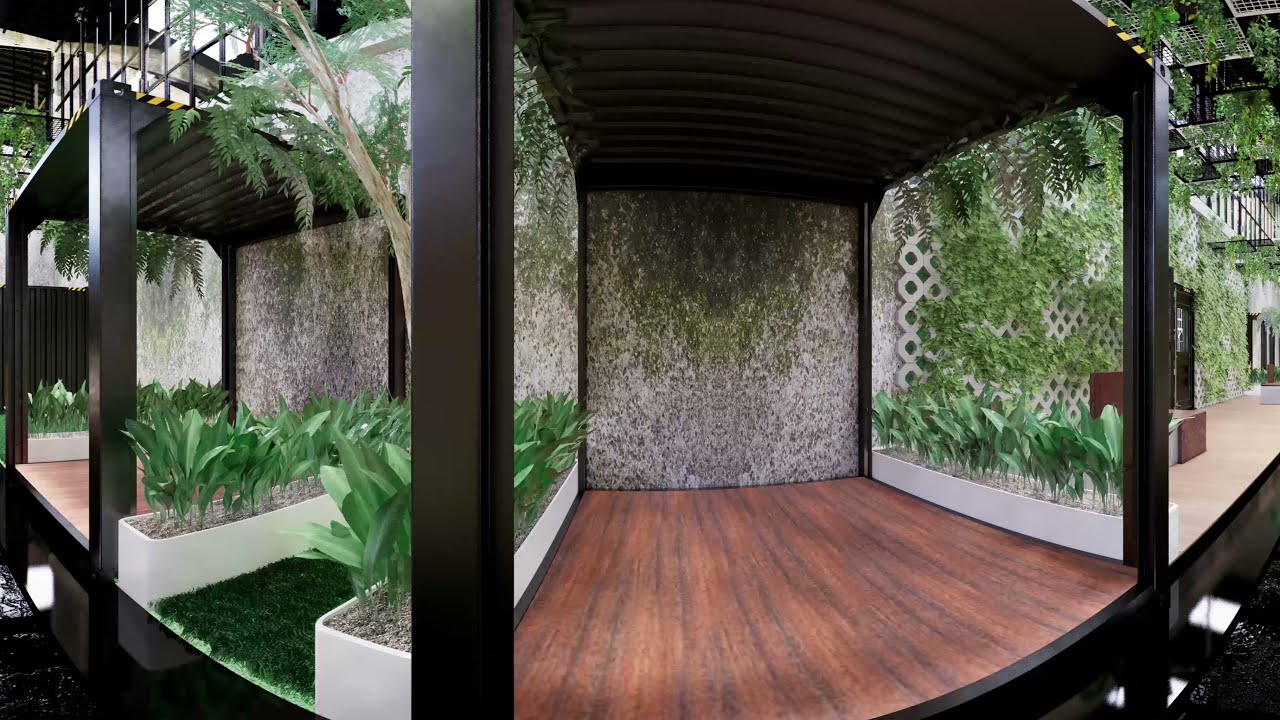The image depicts an outdoor garden patio that could belong to either a residential apartment or a business complex. Dominating the background is a concrete wall adorned with green moss, accompanied by white lattice entwined with a variety of climbing greenery. The patio itself features a wooden floor flanked on both sides by long, white concrete planters brimming with lush, leafy plants. The layout continues with more planters and wooden flooring extending outwards, revealing surrounding balconies and additional greenery. Adding to the structural elements are black columns that ascend to support a possible second level or roof. The visual perspective is slightly skewed, likely the result of a fisheye lens, lending a surreal touch to the composition. The garden is teeming with plants, creating an impression of a verdant, serene haven amidst an urban setting.